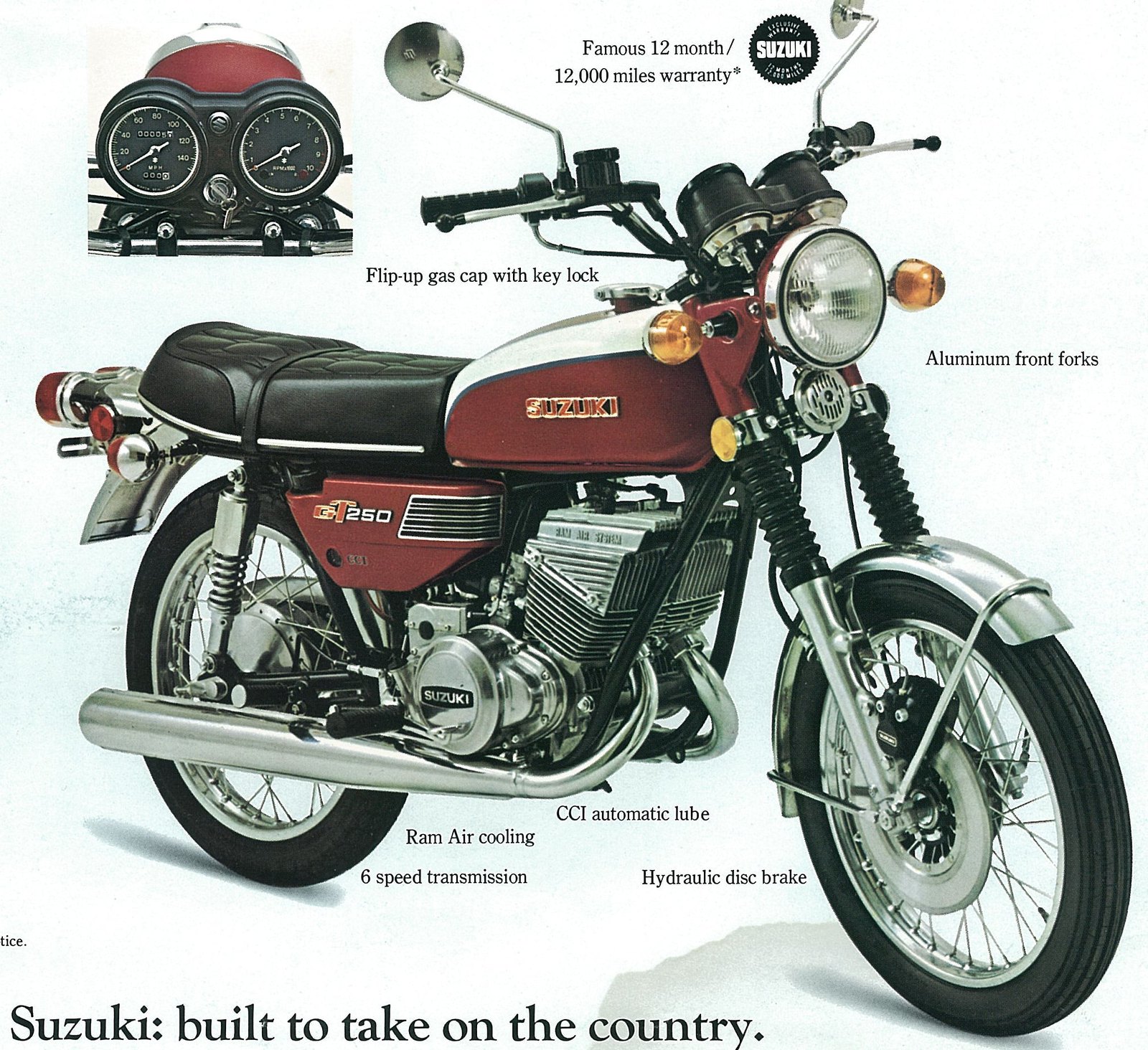This studio photograph showcases a detailed side view of a red and black Suzuki GT250 motorcycle, specifically designed for durability and performance. The image has a white background which highlights the intricate details and labeling of various parts around the motorcycle. Key features include a 12-month/12,000-mile warranty, a flip-up gas cap with key lock, aluminum front forks, CCI automatic lubrication, hydraulic disc brakes, RAM air cooling, and a 6-speed transmission. The top left corner of the image features a close-up of the speedometer settings. The bottom of the image bears the slogan "Suzuki, built to take on the country," encapsulating the robust and adventurous spirit of the bike.